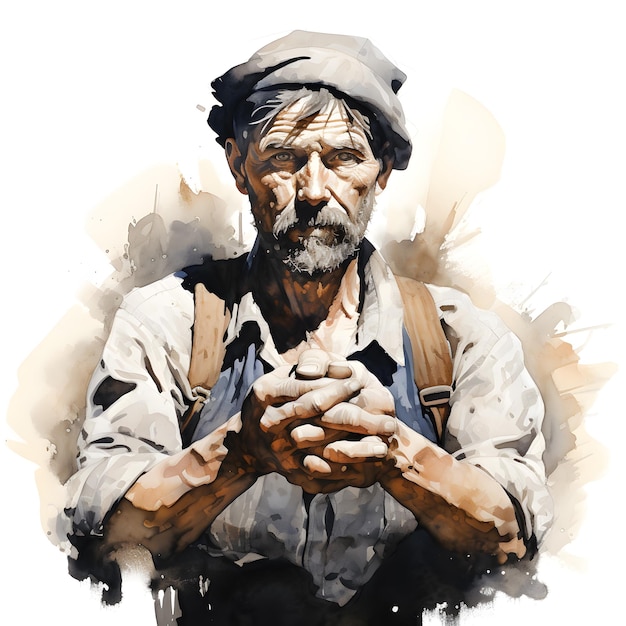This watercolor illustration presents an intense and detailed portrait of an older man, who appears to be a laborer or worker of some sort, possibly a fisherman or woodworker. His face is marked by numerous wrinkles across his high forehead, and his expressive, light-colored eyes convey a pensive look. His beard and mustache are flecked with gray, matching the strands of gray in his black hair that peek out from beneath a worn, gray hat with its brim folded back.

He is dressed in a cream-colored, long-sleeved shirt rolled up to his elbows, showing subtle shades of tan and a worn texture. Over this shirt, he wears what seems to be overalls and the straps of a brown backpack, which sit under his armpits, creating an impression of a life spent in rugged work. His thin frame and sinewy neck muscles emphasize his industrious nature.

The man's hands, clearly work-worn and perhaps arthritic, are clasped in front of him with interlocking fingers, exuding a sense of fatigue and contemplation. His elbows rest on a surface, possibly the armrests of a white or rocking chair, though the full seat is not visible. The background fades into soft tones of gray and mauve, highlighting the man's formidable presence in this evocative piece.